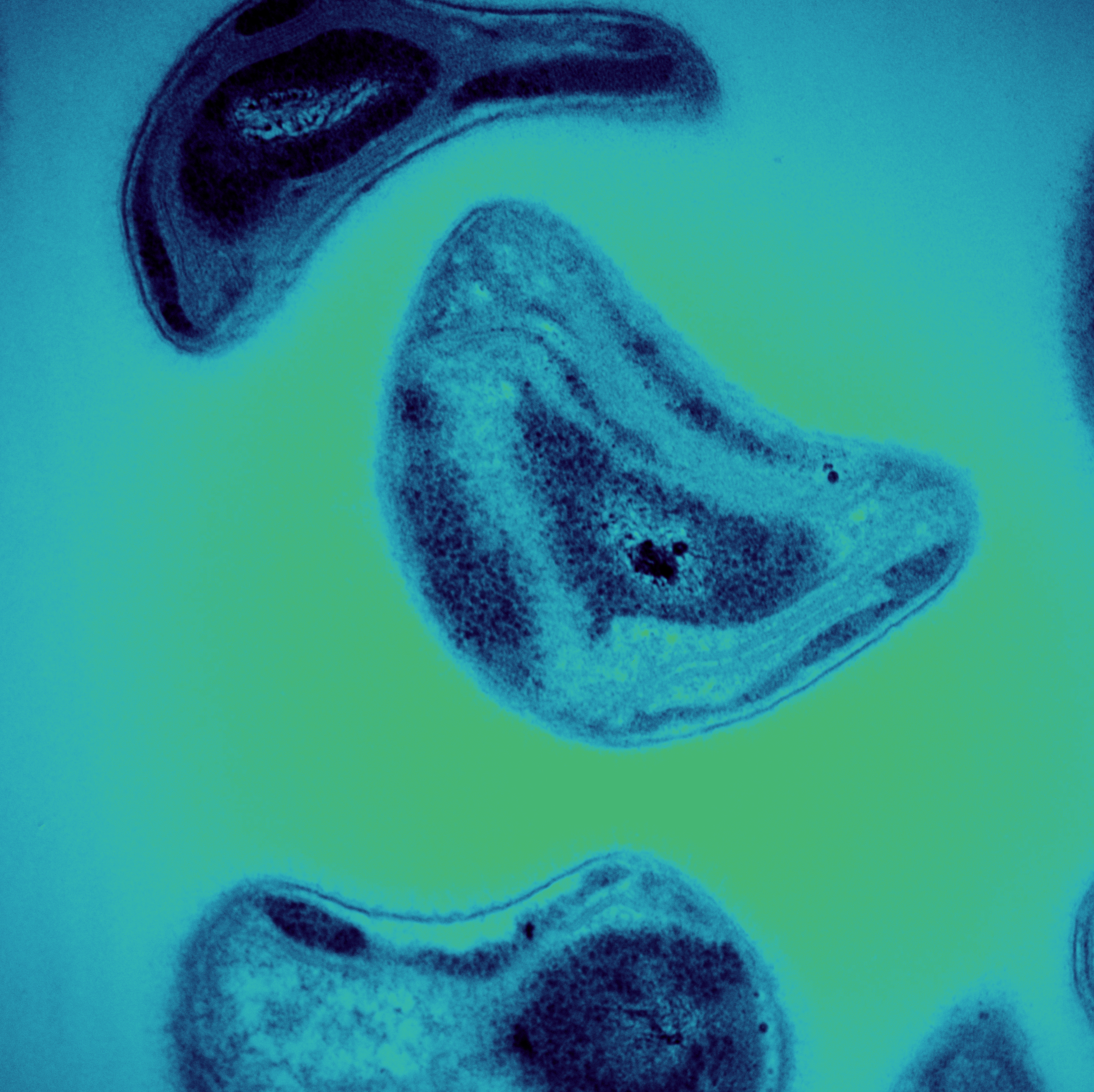The image depicts an abstract view likely captured under a microscope, showcasing a scientific study of cells or microbes. Against a vibrant green background that transitions to a bluish-green toward the edges, several blue-colored shapes are floating, resembling cells or amoeba-like structures. These cells vary in shades, from light blue to dark blue, and their intricate details emphasize the focus on biological or chemical research, although the exact nature of the study remains undefined due to the lack of accompanying text. The scene conveys the exploration of cellular mysteries for scientific purposes, with the cells appearing to drift through their neon-tinted environment.